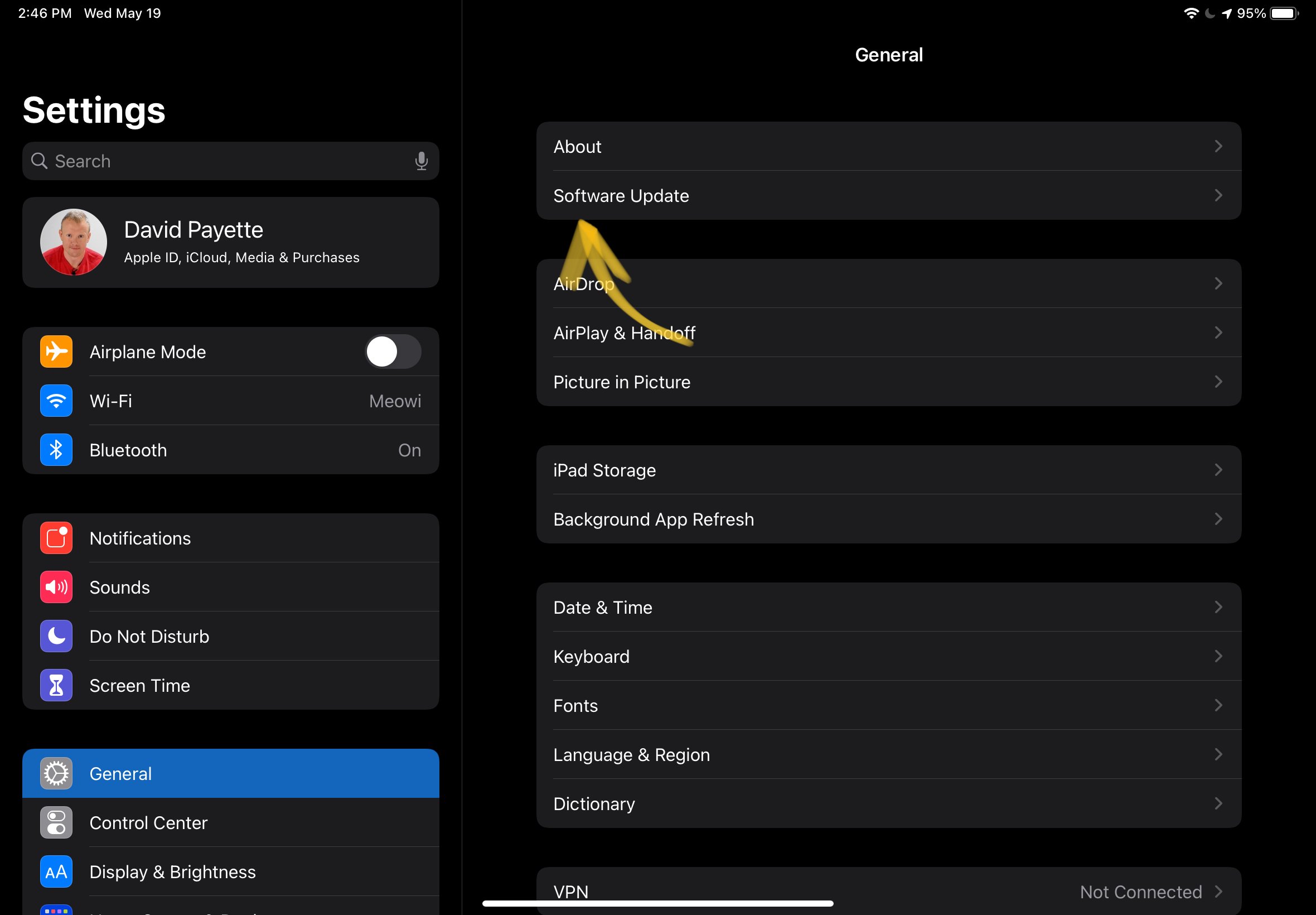Screenshot of a tablet device displaying the Settings menu, with the username "David Payette" prominently shown at the top. The screen showcases a profile picture beside the user's name and includes sections for "Apple ID, iCloud, Media & Purchases". Several options are visible including "Airplane Mode," "Wi-Fi," "Bluetooth," "Notifications," "Sounds," "Do Not Disturb," "Screen Time," and "Control Center." The "General" section is highlighted, and within it, the options "About" and "Software Update" are listed. A green arrow is drawn pointing to the "Software Update" line, indicating where users should navigate to check for software updates. This visual guide aims to instruct individuals on how to access and update their device software.